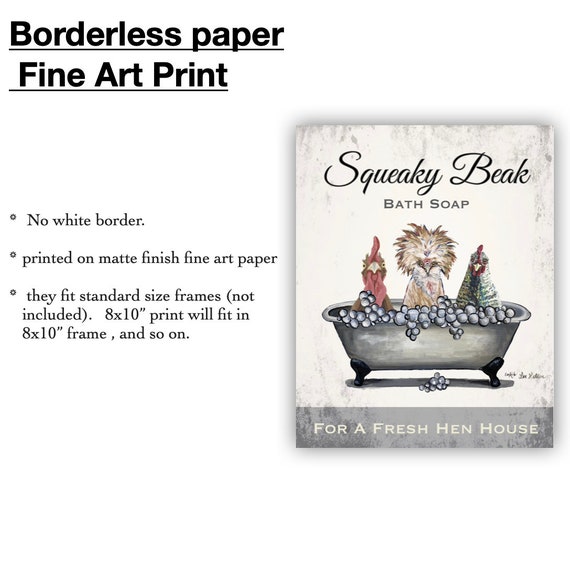The image features an aged, distressed advertisement for "Squeaky Beak Bath Soap" showcasing a whimsical drawing of three quirky chickens, each with distinct features—a red-combed chicken, a brown-bodied chicken with puffy head feathers, and a green-feathered chicken—relaxing in an old-fashioned clawfoot bathtub filled with bubbles, with some bubbles scattered on the floor. The backdrop of the image is primarily white with black edges. To the left, bold text, likely in Helvetica, details the product specifications: "Borderless Paper Fine Art Print," "No white border," "Printed on matte finish fine art paper," and "Fits standard frame sizes; frames not included" (notably an 8 by 10 print). This description is designed to emphasize the fine art print's compatibility with standard frames and the quality of the paper.